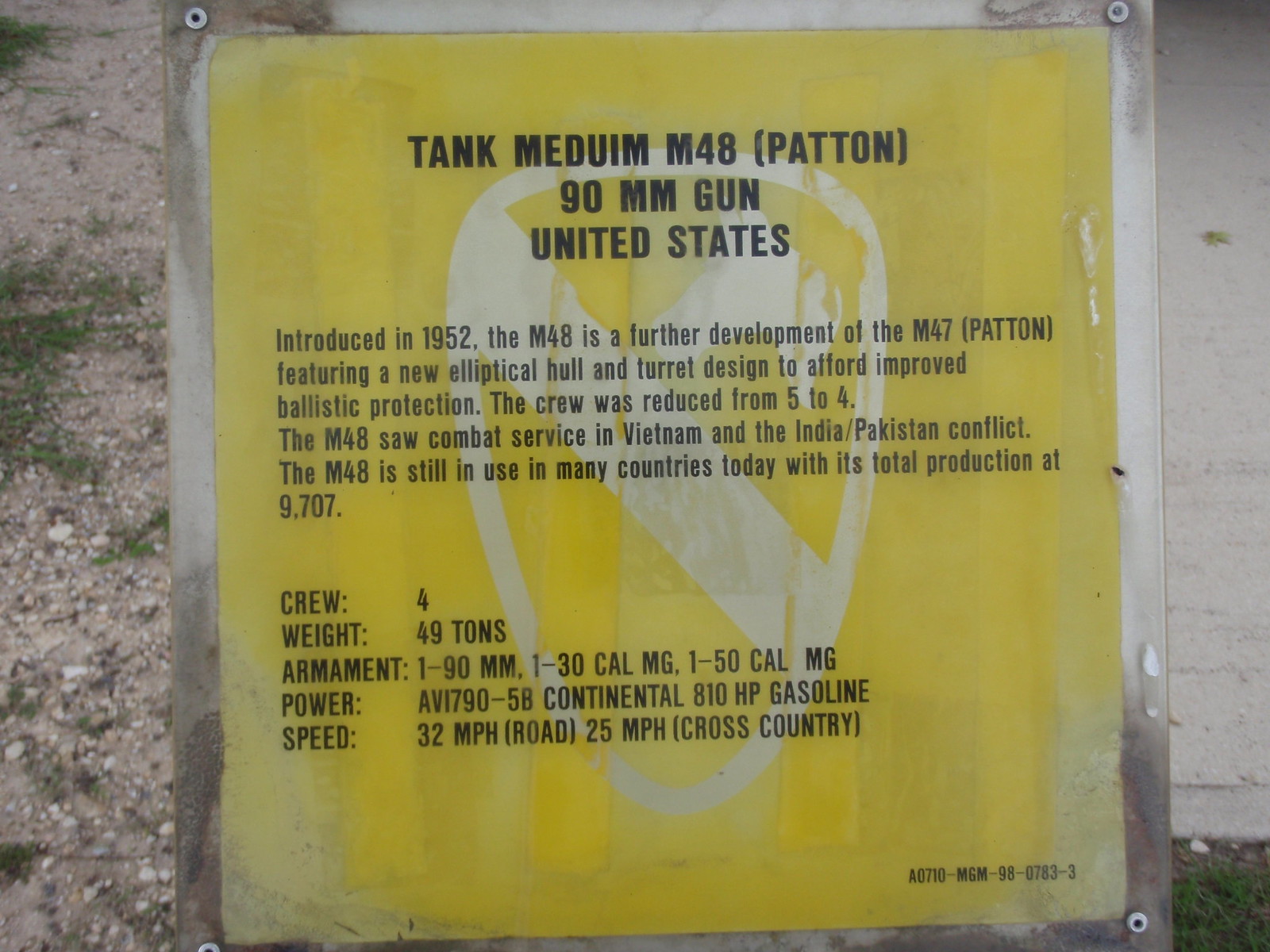This image shows a detailed yellow placard in a metal frame with corner screws, situated likely against a background of ground mixture featuring dirt, rocks, and some grass. The sign is headed with "Tank Medium M48 (Patton)", followed by "90mm Gun" and "United States," all in large black print. The middle section of the placard includes the historical context of the M48 tank, highlighting its introduction in 1952 as an advancement of the M47 Patton, featuring a new elliptical hull and turret designed for improved ballistic protection. Notably, the tank's crew was reduced from five to four members, and it saw service during the Vietnam War and the India-Pakistan conflict. It remains in use in various countries with a total production of 9,707 units. The bottom section lists specifications: Crew (4), Weight (49 tons), Armament (90mm gun, .130 caliber machine gun, .150 caliber machine gun), Power (AVI-790-5B Continental, 810 horsepower gasoline engine), and Speed (32 mph on road, 25 mph cross-country). A white shield with a diagonal sash traverses the sign, adding a distinct emblematic touch.